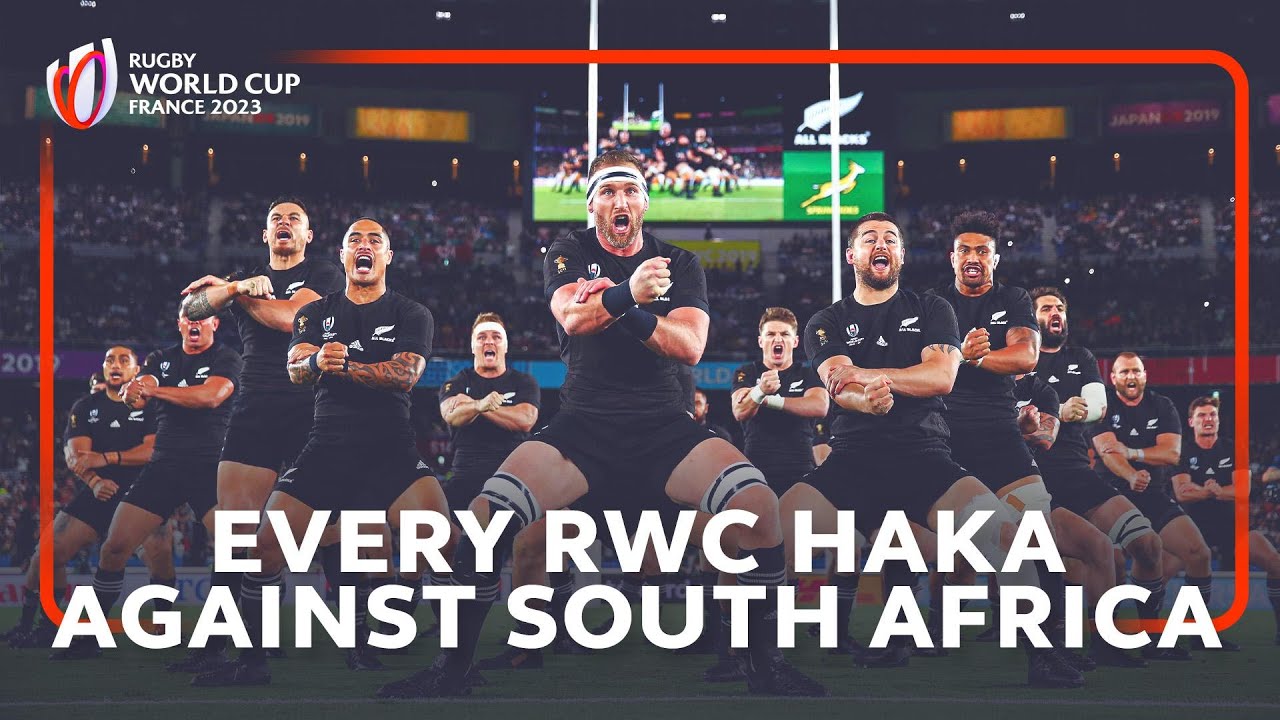The image is a poster advertisement for the Rugby World Cup France 2023, focused on showcasing the traditional Haka performed by a New Zealand rugby team against South Africa. The scene captures approximately 13 men wearing black rugby uniforms, including t-shirts and short, tight-fitting shorts. They are standing in formation with bent knees, arms outstretched, and mouths open, embodying the powerful and emotional display of the Haka. Several of the players are also wearing bandanas or leg bands. Behind them, a blurred stadium crowd and a television screen displaying highlights provide a dynamic backdrop. The top left corner of the image contains the text "Rugby World Cup France 2023" along with a rugby logo. Overlapped across the bottom in bold, white, uppercase letters are the words "Every RWC Haka Against South Africa." The entire scene is framed by a red border, emphasizing its promotional nature.